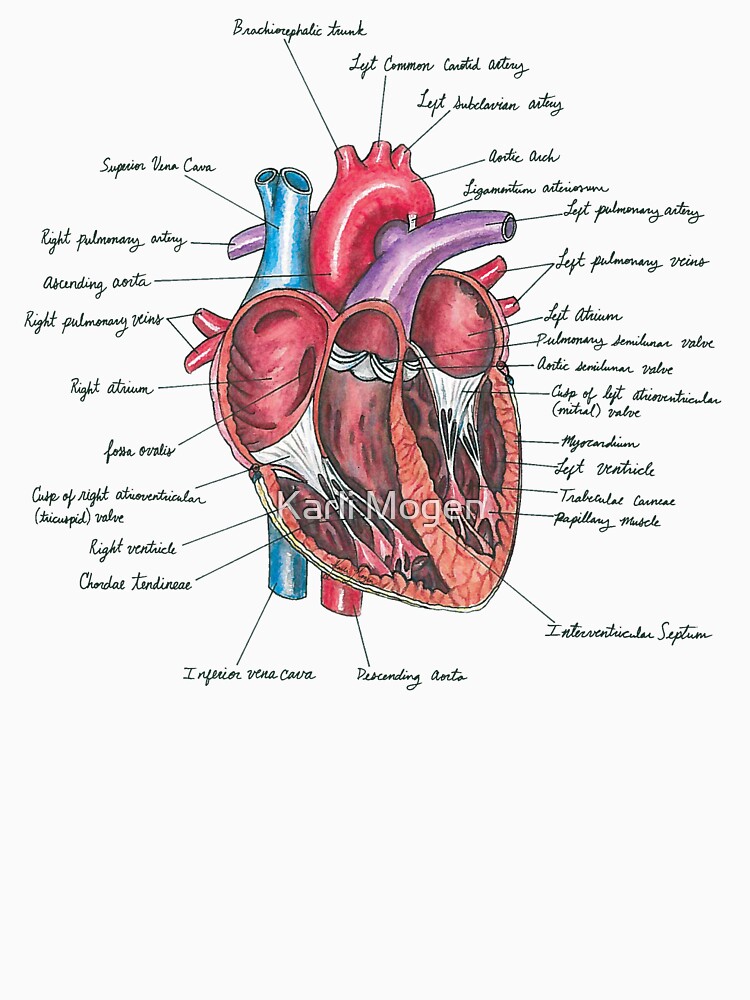The image showcases a highly detailed, anatomically accurate sketch of a human heart. The heart is depicted in color, featuring a variety of hues including red, blue, and purple to differentiate its various structures. The drawing offers a cutaway view, exposing the inner ventricles and chambers, each meticulously illustrated in tones that reflect their anatomical features. The outer walls of the heart are predominantly peach-colored, while the interior is a reddish hue with white, stringy masses connecting several chambers.

Surrounding the heart are numerous handwritten labels in black cursive script, with black lines pointing to specific parts. Key labels include the right atrium, right pulmonary veins, left atrium, and aortic arch, among others. There are over 20 such annotations around the image, detailing parts like the descending aorta, interventricular septum, papillary muscles, and myocardium. Additionally, tubes are illustrated emerging from the heart, including a purple one curving to the right, a blue one standing upright with bifurcations, and a red one with multiple branches.

A watermark reading "Carly Mogen" is positioned in the middle of the picture, serving as a signature.